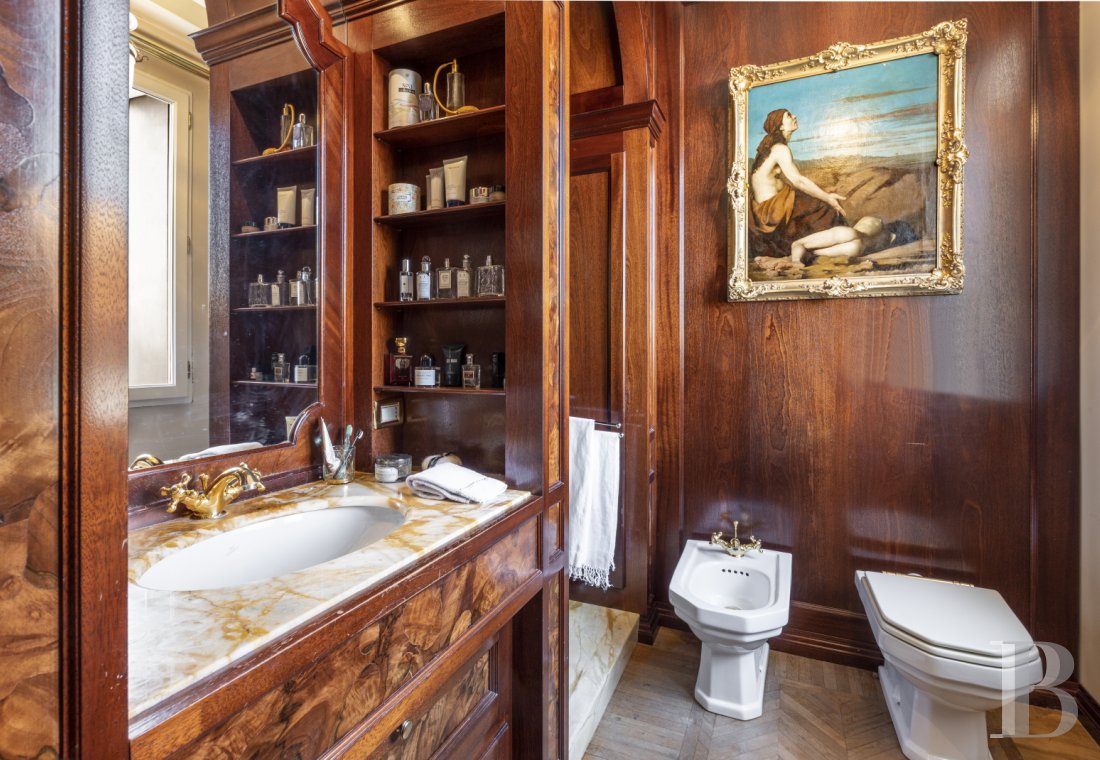The image depicts an ornate and vintage bathroom adorned with dark, shiny wood paneling on the walls and hardwood flooring. The focal point on the left side is a sink featuring a marble countertop with intricate gold leaf details and a gold faucet. Positioned nearby are wooden shelves integrated into the paneling, holding various bottles, colognes, and lotions, with drawers and cabinets below.

In the center, there's a white porcelain toilet next to a bidet, with white towels hanging nearby. Adjacent to that is an open shower, partially visible. Above the toilet hangs a distinctive gold-framed photograph portraying a woman gazing up at the sky, accompanied by another woman lying on the ground.

The bathroom, potentially a highlight for a design site, showcases a mix of luxurious materials and a classic aesthetic not commonly seen today.